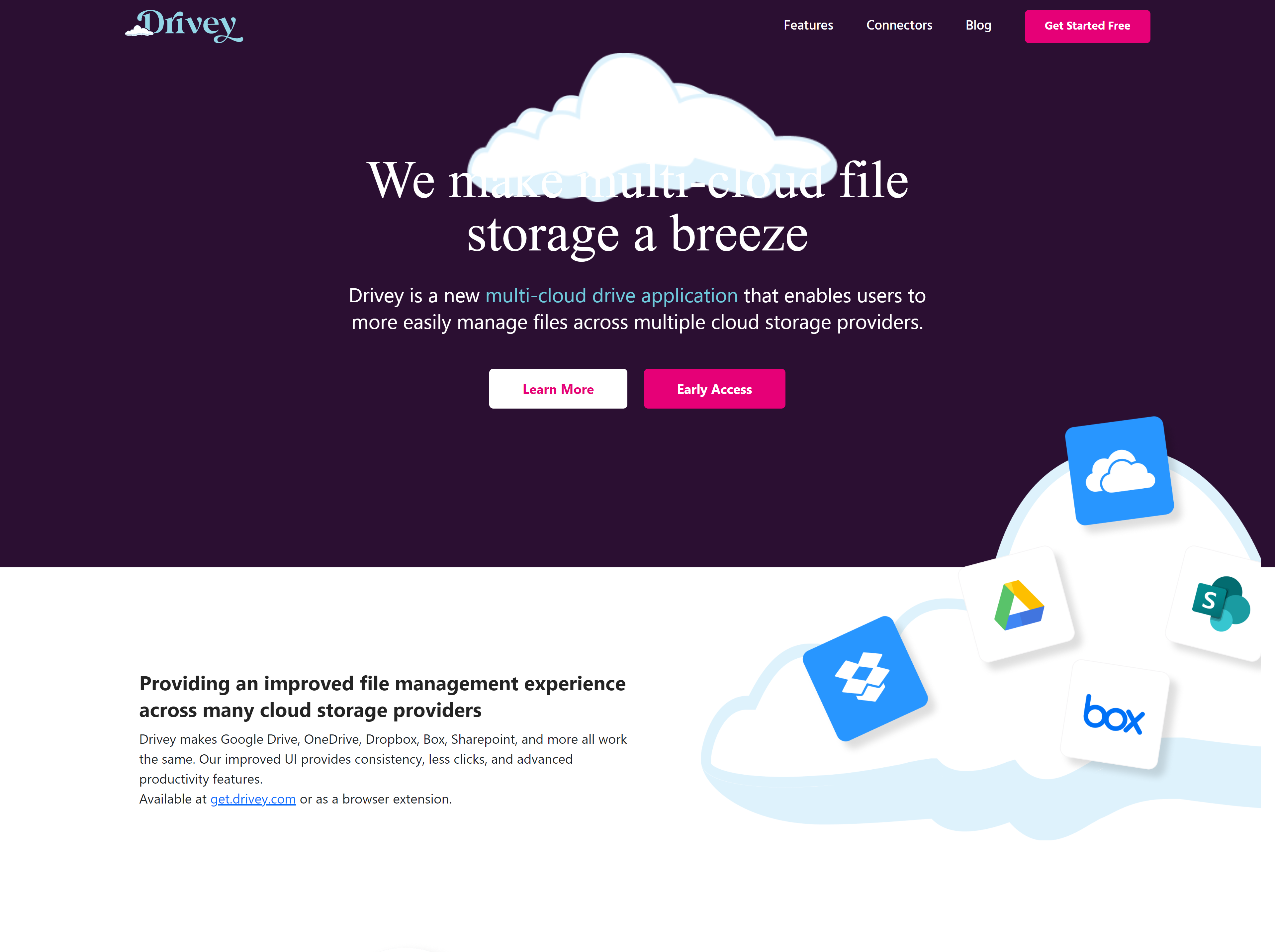The image highlights the Drivey website, with its name displayed prominently at the top left. At the top right, there is a pink button labeled "Get Started Free" in white text. To its left are three navigation categories: Blog, Connectors, and Features. Centrally positioned at the top, it reads, "We make multi-cloud file storage a breeze," overlaid on a cloud graphic, all set against a dark purple background.

In the middle of the image, the text introduces Drivey as a new multi-cloud drive application that simplifies file management across multiple cloud storage providers. Below this description are two actionable buttons: "Learn More" on the left, and "Early Access" on the right.

At the very bottom left, the image elaborates on Drivey's benefits, stating: "Providing an improved file management experience across many cloud storage providers, Drivey makes Google Drive, OneDrive, Dropbox, Box, SharePoint, and more all work the same. Our improved UI provides consistency, fewer clicks, and advanced productivity features. Available at GetDrivey.com."